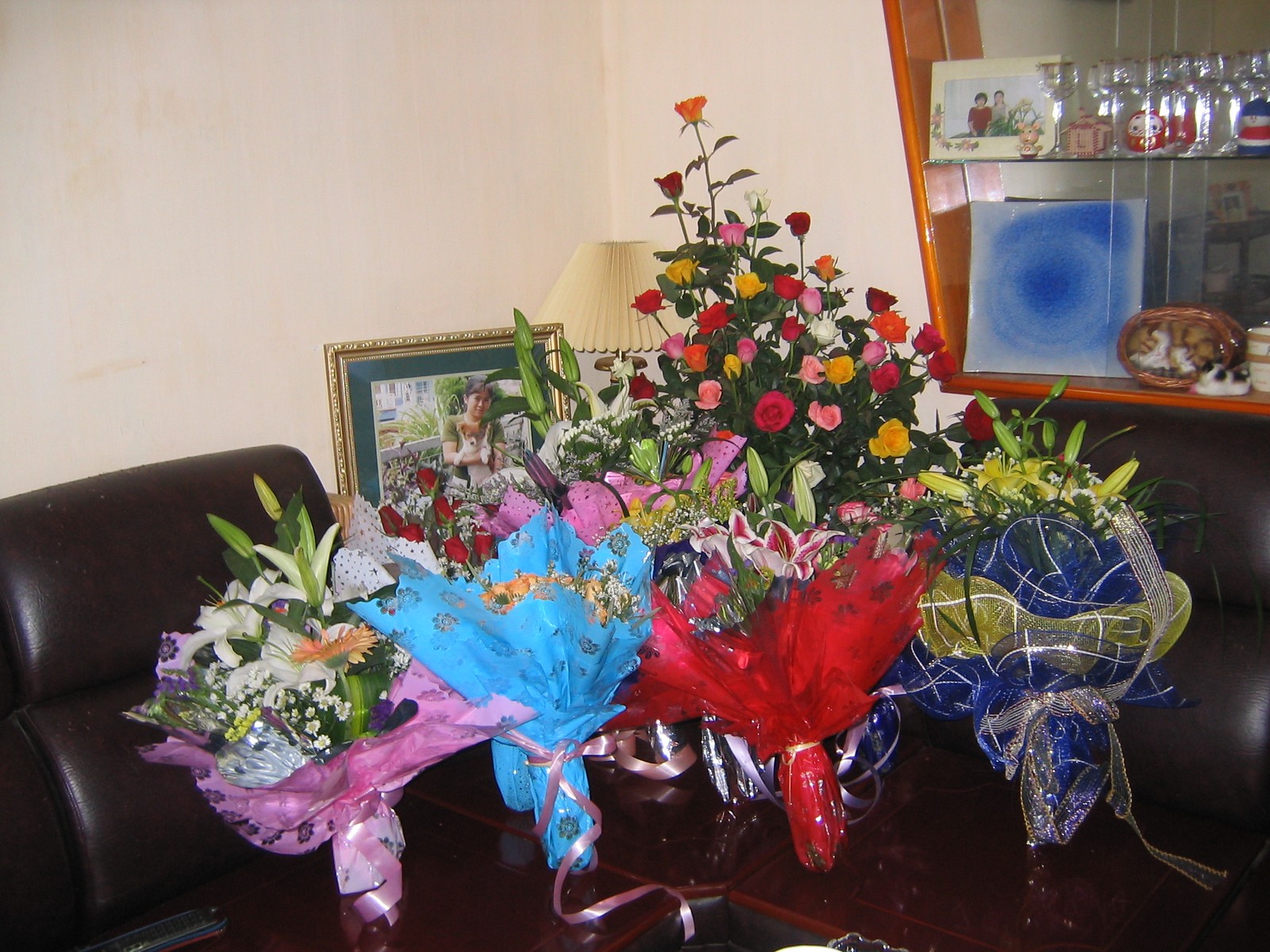The photograph depicts a room filled with an array of intricately arranged floral bouquets, showcasing a range of vibrant colors and textures. From left to right, the floral display begins with a bouquet wrapped in purple paper, featuring a harmonious mix of white, orange, purple flowers, and baby's breath, secured with a pink bow. Adjacent to it is a blue-wrapped bouquet adorned with red roses and baby's breath, tied with another pink bow. Next is a striking bouquet wrapped in red paper with a yellow bow, containing pink and red flowers. Farther right, another bouquet, held together by navy blue material with white stripes and a silver and yellow bow, features tall yellow flowers interspersed with unopened buds and green foliage. Behind this main row, towering multicolored roses in hues of yellow, red, pink, and orange are visible, adding to the rich tapestry of the display.

The flowers are meticulously placed on a dark wood, shiny table, beneath which is a burgundy-colored chair, presumably vinyl or leather. The room itself is softly lit by a lamp with a beige lampshade. A focal point in the background is a framed portrait of a dark-haired woman or young girl holding a brown and white dog, set against a backdrop of a building and a tree. The frame is dark turquoise with a gold border. The back wall is painted in a soothing beige tone with subtle hints of darker tan. Adjacent to the floral arrangements, a wooden shelving unit with mirrored glass houses various clear glass items, a white plate with a blue center, and possibly a figurine of a cat. This carefully curated composition suggests that the flowers might be a tribute to someone who has recently passed away, perhaps the person in the portrait, creating a somber yet beautiful scene.